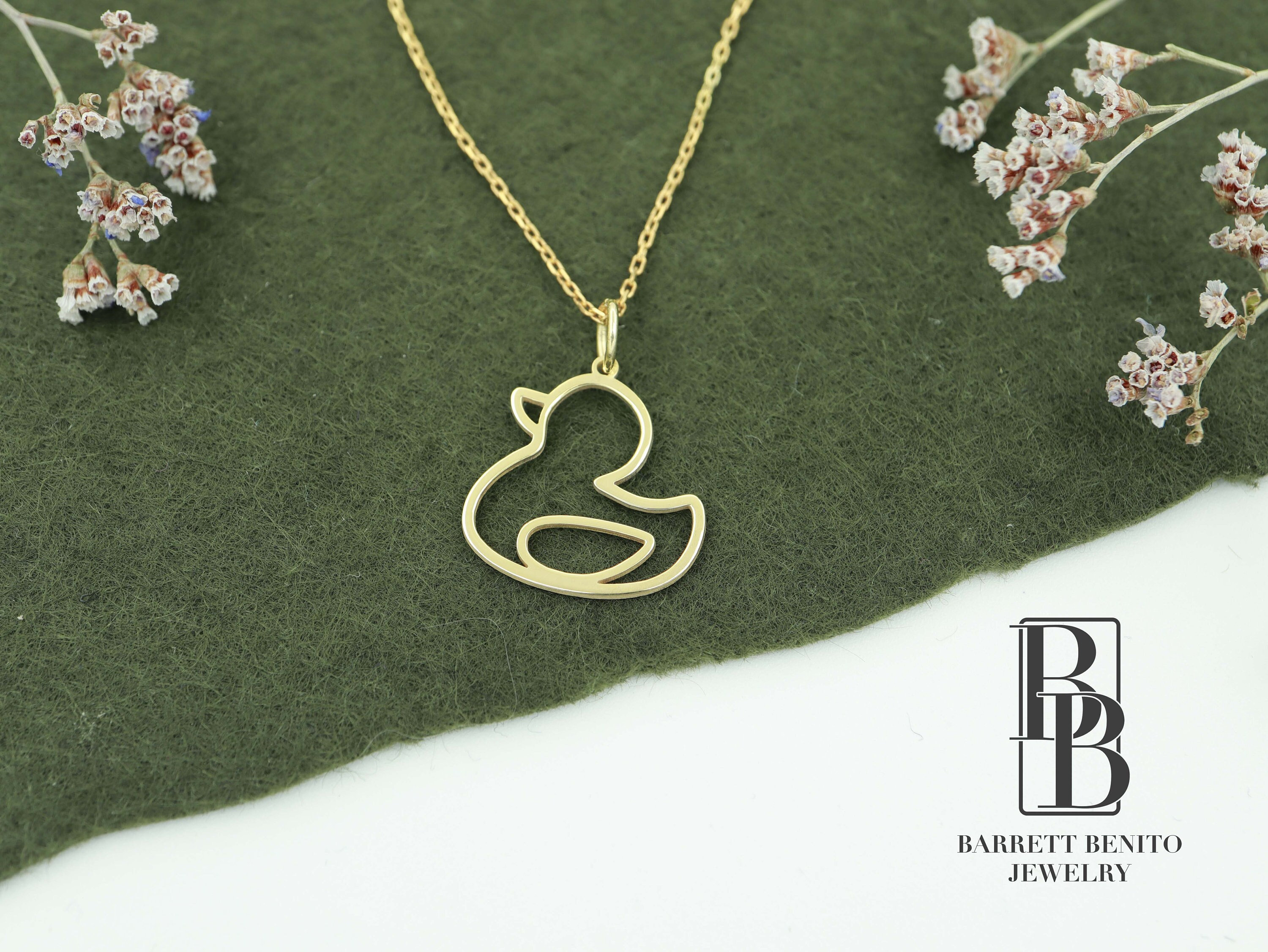This photograph features a gold necklace prominently displayed against a contrasting background. The necklace, crafted by Barrett Benito Jewelry, consists of two delicate gold strands meeting at a centerpiece—a simplistic yet elegant golden pendant shaped like an abstract outline of a duck. The duck pendant, resembling a rubber duck, includes discernible features such as the beak, wing, tail, and head, but in a minimalist design. The necklace is artistically laid out on a green, shaggy felt background, which transitions into a white area toward the bottom of the image. Flanking the necklace on both sides are small branches of white flowers, adding a decorative touch to the display. In the lower right corner, set against the white background, is the black rectangular logo of Barrett Benito Jewelry, featuring two uppercase B's stacked vertically. The meticulous arrangement of the necklace and flowers creates a visually appealing and sophisticated presentation.